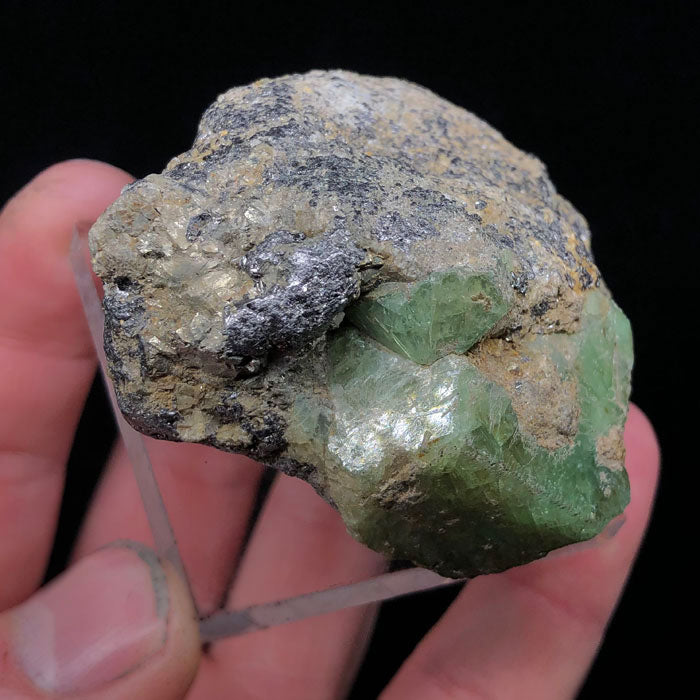In this striking image, a Caucasian man's hand is prominently displayed against a completely black background, showcasing a fascinating mineral rock. The hand, with visible dirt under the thumbnail, holds the rock sample securely, positioned on a square piece of clear acrylic glass and supported by two thin silver brackets. The rock itself, primarily gray, is adorned with vibrant green and golden crystal flakes. The left side of the rock features interlaced silver and whitish crystals, while the right side is dominated by green, emerald-like gemstone colorations with a hint of brown. The close-up shot emphasizes the rough yet intricate textures of both the hand and the extraordinary rock specimen.